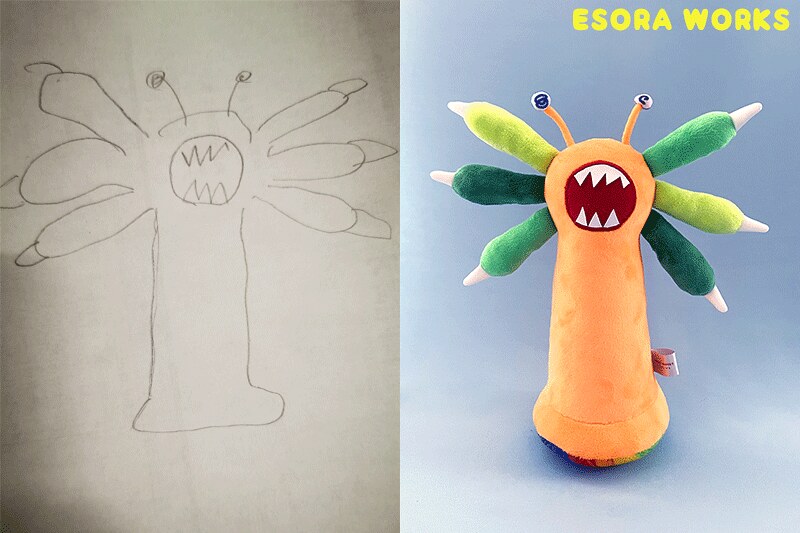In this split-screen image, we see a side-by-side comparison of a pencil drawing and its fabric recreation. On the left, there's a rudimentary black-and-white pencil sketch on white drawing paper, depicting a whimsical creature with a round head adorned with googly blue eyes on extended stalks, a wide open mouth filled with jagged teeth, and six varied green tentacles, resembling an amoeba. The drawing appears youthful and simple, likely done by a child. On the right, the sketch has been brought to life as a plush toy labeled "Isora Works" (misread as "Essura Walks" in yellow text above the creature). This colorful representation features an orange body, the same protruding eyes, tentacles with white spikes, and a big, toothy mouth. The toy closely mirrors the drawing while giving it a playful and tangible dimension, complete with an unreadable tag on its side.